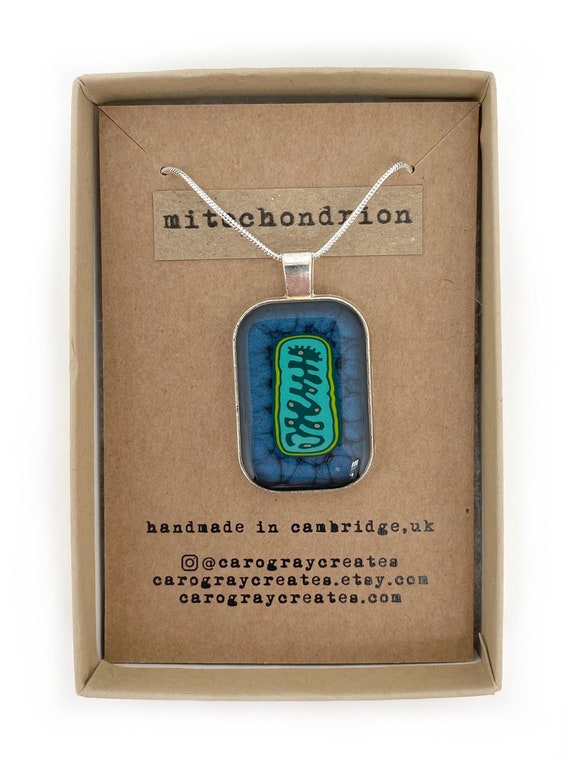The image depicts a close-up view of an open brown cardboard jewelry box set against a white background. Inside the box, there is a cardboard holder displaying a necklace. The necklace consists of a silver chain attached to a pendant, which has a rectangular shape with curved corners. The pendant's design features an abstract, dark, sunflower-like shape from top to bottom, with blue and greenish-blue interior colors and a dark, almost black, outline. In the center of the pendant, there's a gemstone that resembles an eye in a blue color. Above the pendant, "Mitochondrion" is written in black text. Below it, the box displays text in black letters that read, "Handmade in Cambridge, UK." Additionally, it includes social media and website information: "@CarlGrayCreates," "CarlGrayCreates.etsy.com," and "CarlGrayCreates.com."